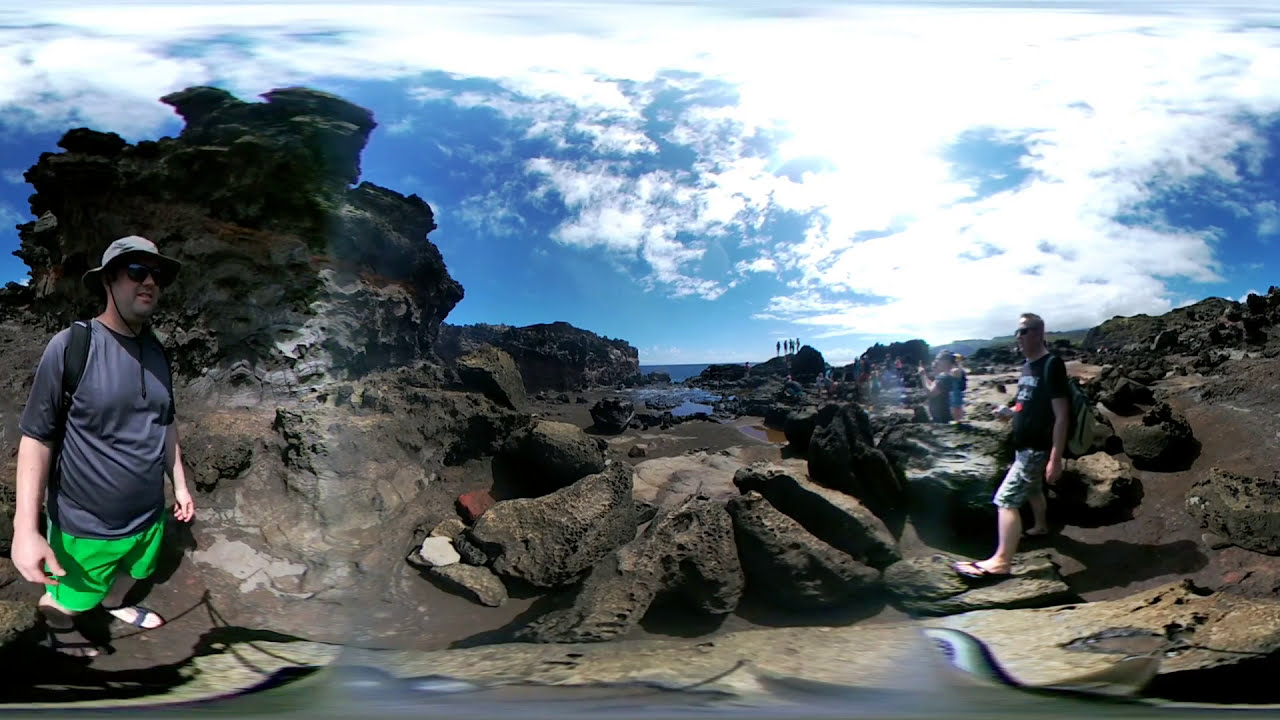The photograph captures an outdoor scenic moment at a rocky beach under a blue sky with white clouds. In the foreground, there are two men walking along the rugged coastline. The man on the left is wearing a white wide-brim cap with darker markings, dark sunglasses, a gray t-shirt, lime green shorts, and black sandals. He has black straps over his shoulders, likely from a backpack. The man on the right is dressed in a black t-shirt with white writing and something red on its front, light-colored shorts, black sandals, and dark sunglasses, with his head slightly turned towards the camera. In the middle of the image, the craggy terrain features pools of water among the rock formations, giving way to the ocean in the distance. Perched atop one of these large rocky outcrops is a small group of about five people, possibly hikers, their silhouettes distinct against the backdrop of the expansive, partly cloudy sky. The setting appears to be a panoramic coastal landscape filled with a mix of sand and rocky outcroppings.